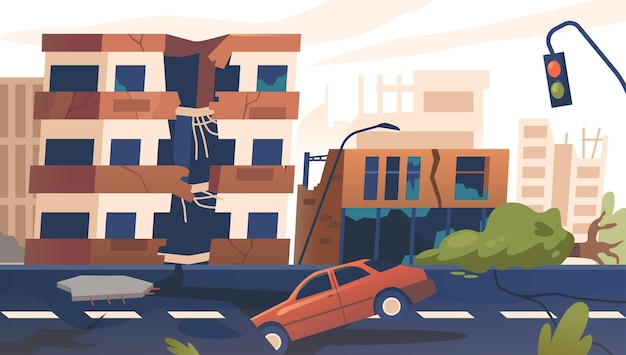The image is a detailed cartoon-style drawing of a devastated cityscape, primarily showcasing muted tones of white, coral, and warm orange hues. In the background, a rudimentary three-story building with light and dark tan highlights stands on the left, visibly split down the middle with exposed rebar and hanging wires, hinting at severe earthquake damage. To the right is a shorter, squatter building, also ravaged by cracks, with four broken windows. Uprooted trees lie horizontally in front of the buildings, adding to the scene's chaos. A bent streetlamp post towers above, displaying only green and red lights. The foreground features a black road with a white dotted line down the center, fissured by a significant crack. An orange car's front bumper and tire are precariously lodged in this gap, propping the vehicle at a diagonal angle.